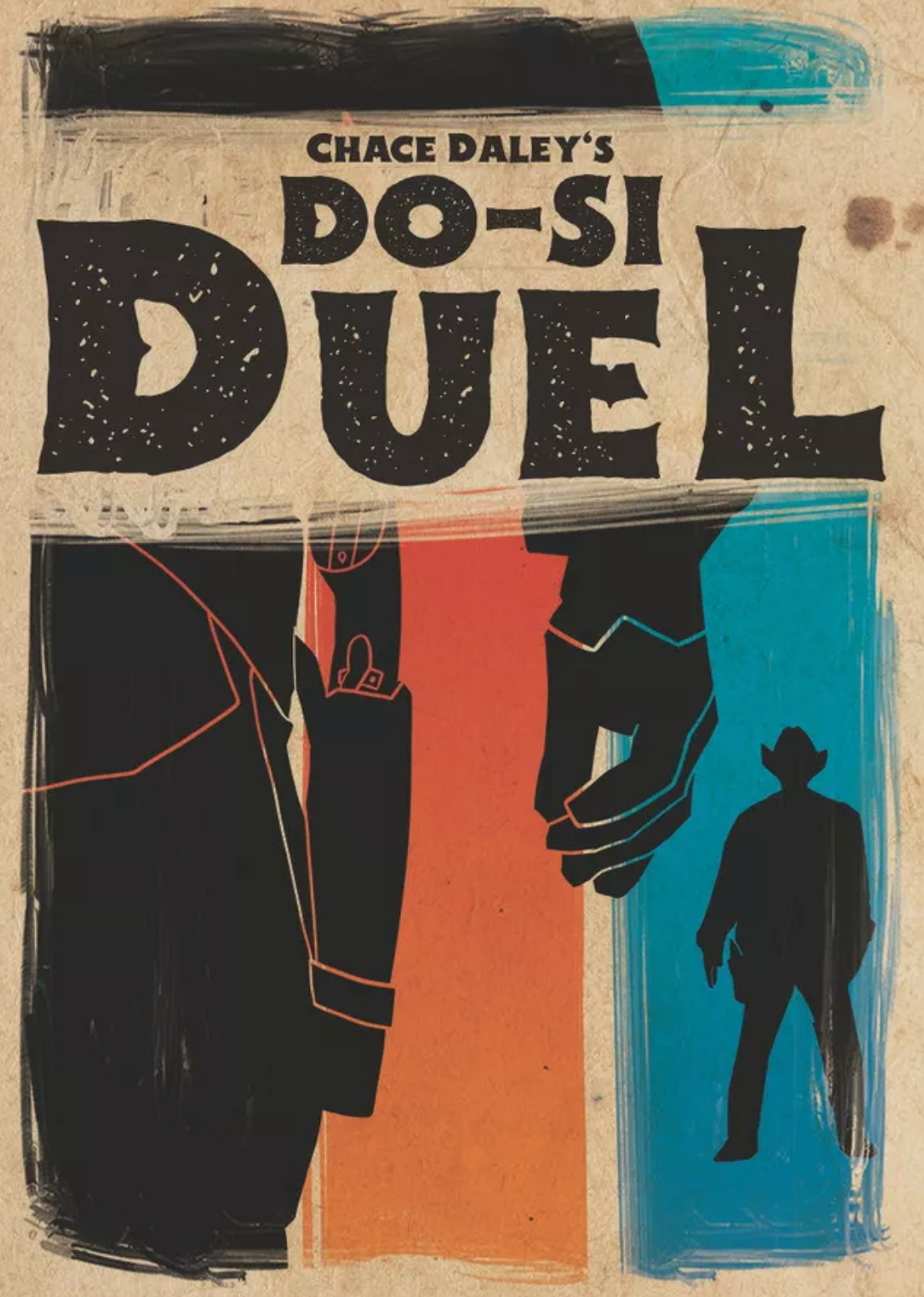The image appears to be a book cover or potentially a movie poster with a distinctly Western theme. The title, "Chase Daly's Doocy Duel," is prominently displayed in large, bold black Western-style text. The backdrop features two contrasting streaks of color—a red streak in the center and a blue streak to the right—creating a dynamic visual effect. The scene is dominated by two black silhouettes of cowboys: one in the foreground, shown from the back with just the right side visible, including his hand near the pistol at his hip, a perspective that feels as if the viewer is standing right behind him. The second cowboy is positioned farther away, his full silhouette visible with his hand poised near his holstered pistol, indicating an imminent duel. The overall artistic style combines elements of both pencil and paintbrush, lending the image an old, worn appearance.